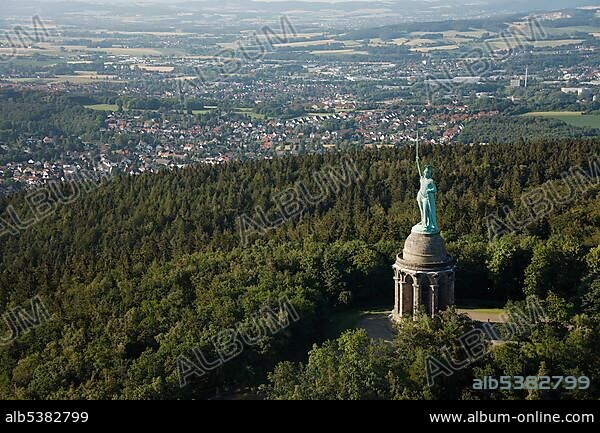The image is a photograph reminiscent of a postcard, marked diagonally from the lower left to the upper right corner with "Album" in a white outlined watermark. At the bottom left corner, an identifier reads "ALB5382799," and in the bottom right corner, the website "www.album-online.com" appears. The foreground features a temple-like monument with a domed roof and columns supporting the base. Standing atop the dome is a statue of a man with a greenish patina, dressed in flowing robes, his right arm extended upwards with a sword. Surrounding this structure is a lush, heavily wooded area on a hill or mountain. In the background, a vast plain stretches out, showcasing a patchwork of green fields and a sprawling cityscape composed of white and red-roofed houses, farms, and various buildings.